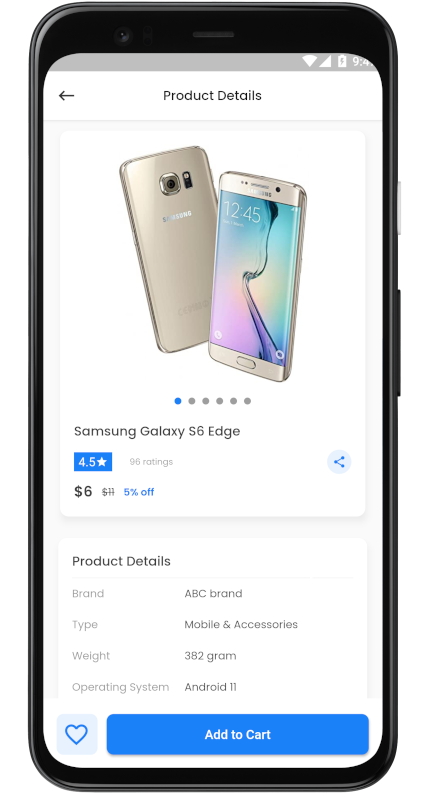A detailed photograph of a Samsung Galaxy cell phone is displayed, showcasing the entire device from edge to edge. The phone's screen features a frozen webpage, presumably a product information page for a Samsung Galaxy S6 Edge. At the top of the screen, a gray status bar displays standard cell phone icons including signal strength, battery life, and the current time. 

Below this, a white rectangular navigation bar spans the width of the screen. Within this bar, a back arrow is present alongside the text "Product Details." Directly below, the screen presents an image of both the front and back of a Samsung Galaxy S6 Edge. The description "Samsung Galaxy S6 Edge" is prominently displayed beneath these images.

Further down, a rating box reveals that the phone has garnered 4.5 stars from 96 reviewers, indicative of generally high user satisfaction. Additional product details follow, listing the brand, item type, weight in grams, and operating system of the phone. Finally, an "Add to Cart" option is visible, inviting users to purchase the device directly from this page.